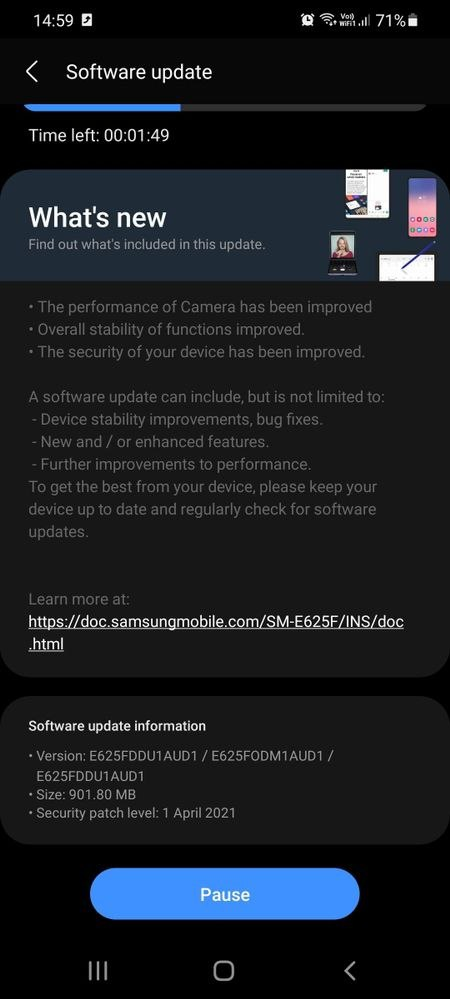This image showcases a software update notification on a mobile device in dark mode. The interface is set against a black background and displays various standard icons in the notification bar at the top, including the current time (14:59), data connectivity, Wi-Fi, alarm clock, and a 71% battery icon.

In the top-left corner, there is a back arrow symbol indicating the option to return to the previous screen. Beneath it, the text "Software Update" is prominently displayed, with a progress bar below that is approximately one-third filled in blue, showing "Time left: 00:01:49."

A section titled "What's New?" is present, accompanied by several tech-related images on the right side. The update details below this section include:

- **Enhanced Camera Performance**: Improvements to the functionality and quality of the camera.
- **Overall Stability Improvements**: General enhancements to the stability of device functions.
- **Security Enhancements**: Upgraded security features to better protect the device.

Further information states that software updates may include device stability improvements, bug fixes, new or enhanced features, and more performance improvements. Users are encouraged to keep their devices up-to-date to benefit from these enhancements and are directed to "Learn more at https://doc.samsungmobile.com/sme625f/ins/doc.html."

The device's software update version numbers E625FDDU1AUD1 / E625FODM1AUD1 / E625FDDU1AUD1, the file size of 901.8 MB, and the security patch level dated 1 April 2021 are also listed. A blue pause button is visible at the bottom of the screen.